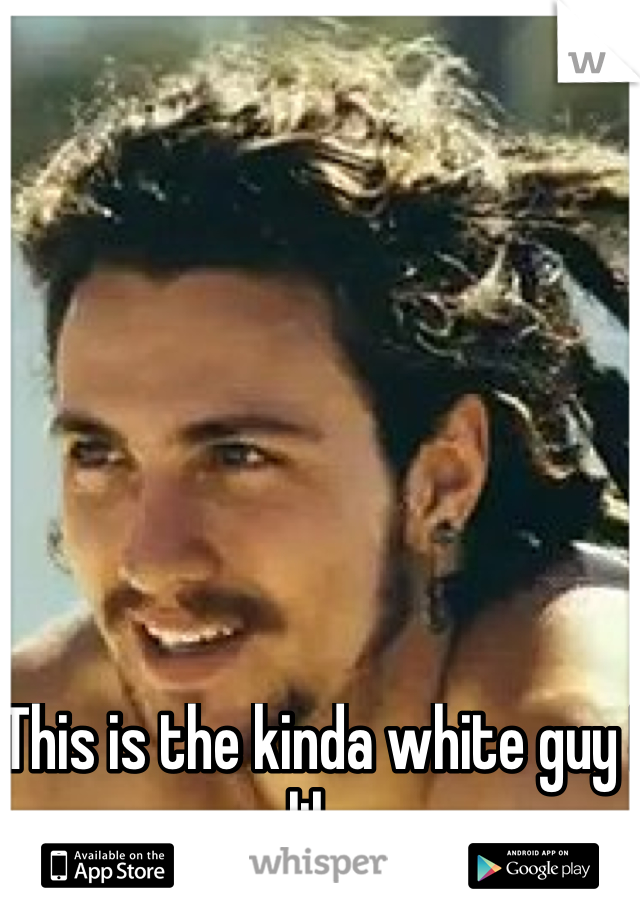The image is a detailed, close-up photograph of a Caucasian man with dark brown, long, wavy hair that appears unkempt, resembling a rat's nest, and is pulled back with a slight widow's peak. He has dark brown eyes, thick eyebrows, and dark long earrings. The man sports a moustache and a beard that extends to long sideburns, potentially forming a goatee. He is not looking directly at the camera but gazing off to the side, with a slight smile on his face. Beneath his chin, in white text, there's a partially visible quote that begins with "this is the kind of white guy," suggesting a humorous or mocking tone. Below the image, there are icons indicating availability on the App Store and Google Play, with the word "Whisper" in lowercase letters in the center, hinting that this image is likely an advertisement for the Whisper app.